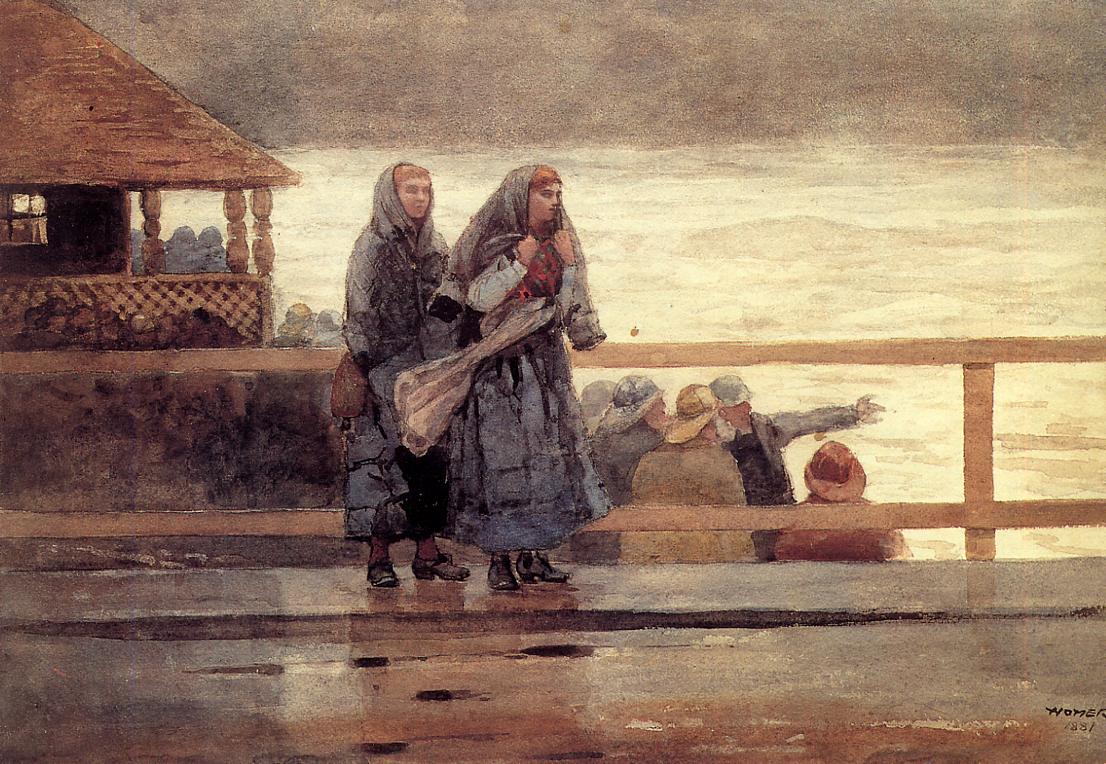This horizontally aligned oil painting, characterized by its blurry, impressionistic style, depicts a somber, cold scene featuring two women overlooking a dull, gray body of water. Both women are clad in matching blackish-gray gowns and black shoes, with gray headscarves partially covering their reddish-brown hair, tufts of which poke out. One woman is seen clutching her headscarf. The women are standing on what could be a brown wooden or stone platform, possibly a bridge, dock, or street, next to a wooden fence. Below the fence, a group of fishermen, adorned in rain jackets and hats of varying colors such as yellow, red, and blue, gathers, with one man gesturing toward the water. The murky water is represented through horizontal strokes of white, light gray, and brown. In the far left corner, a brown house with a porch and roof is partially visible. The overall palette of the painting includes shades of black, white, gray, tan, brown, blue, and some red, emphasizing its cold, dreary atmosphere. Lastly, an indistinct black scribble in the bottom right corner hints at the possible signature "Homer 1881."